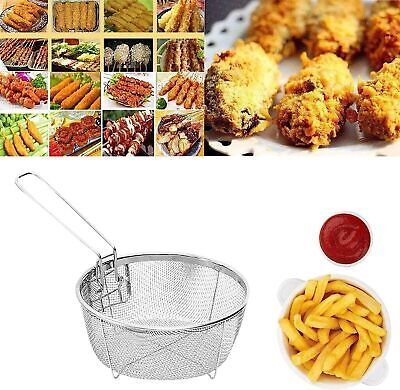The image is a multi-sectioned poster displaying various types of fried foods. The top half of the poster is divided into two sections: on the right, there is a photograph featuring what appears to be fried jalapeno poppers. The left section is a 4x4 grid collage comprising 16 smaller photographs of different fried snacks, including corn dogs and possibly some sweet foods. The bottom half of the poster has a circular fryer basket with a handle typical of standard fryer baskets. To the right of the basket is a white bowl with small half-circle handles containing french fries, and just above the bowl is a small cup of what looks like ketchup.